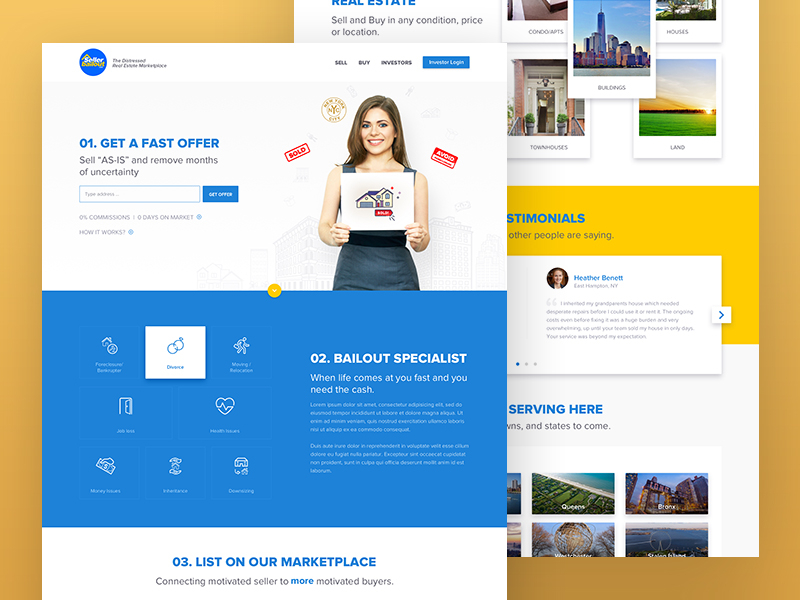This image from a website advertises a real estate service that specializes in buying homes in any condition, at any price, and in any location. The image features a smiling woman, around 35 years old, holding a piece of paper with a drawing of a house with a garage. She exudes confidence and happiness. The website offers a quick and hassle-free way to get an offer, allowing sellers to bypass months of uncertainty by selling their homes "as is." Below the image, a caption reads: "Bailout Specialist: When life comes at you fast and you need the cash." Additional visuals include pictures of a city by the water and open land, along with testimonials from satisfied customers. The service also highlights a unique feature: listing on their marketplace to connect motivated sellers with even more motivated buyers.